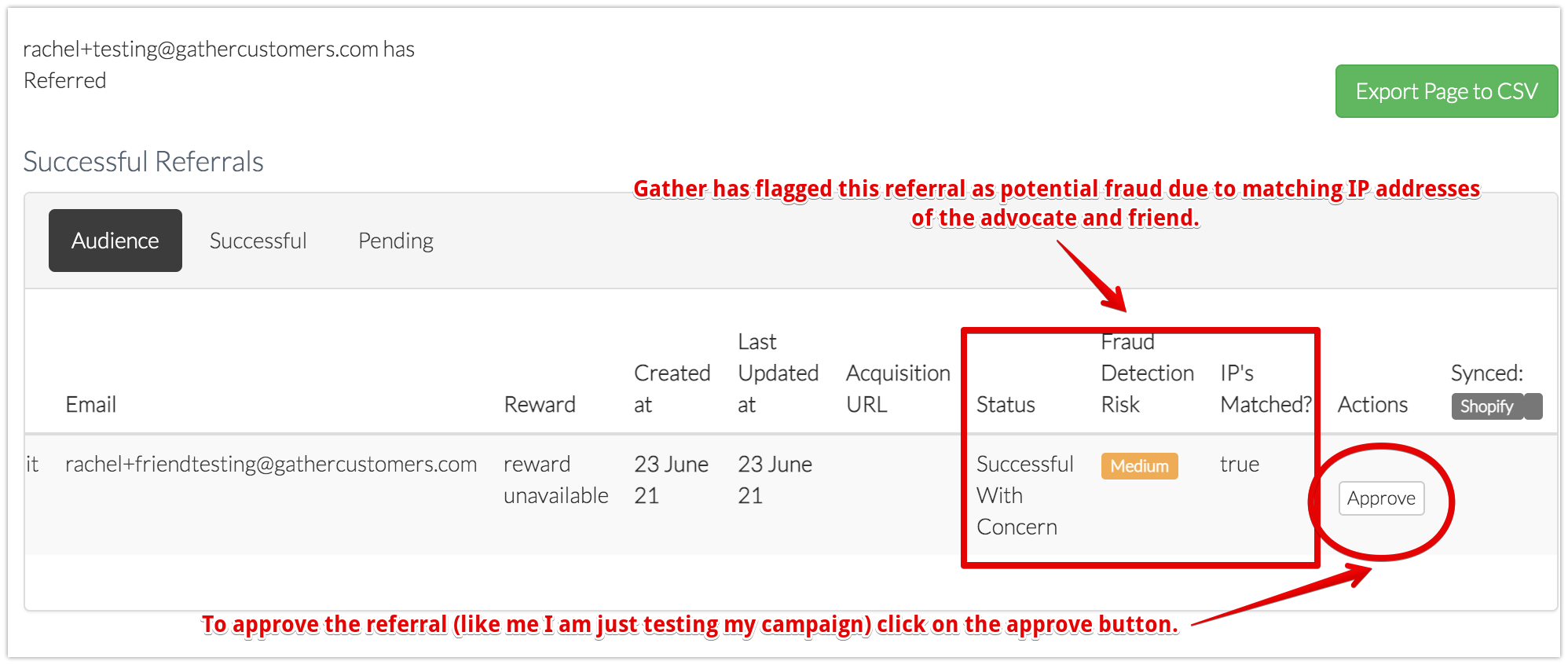The image depicts a software testing field for an email referral system, specifically for the email address raquelplus.testing@gatheredcustomers.com which has been flagged for potential fraud. The interface includes a variety of data fields and options, with a distinct green button located in the upper right corner for exporting data to a CSV file (comma-separated values).

At the top of the screen, the user can toggle between different views: "Audience", "Successful", and "Pending", with the "Audience" option currently selected, indicated by a gray rectangle around it. Below this, several headers structure the referral data: "Email", "Reward", "Created At", "Last Updated At", "Acquisition URL", "Status", "Fraud Detection Risk", "IP is Matched?", and "Actions". The details under these headers display an entered test email, raquelplus.testing@gatheredcustomers.com. The "Created At" and "Last Updated At" dates are in a stacked format, as are the "Acquisition URL", "Status", "Fraud Detection Risk", and "IP is Matched?" fields.

The data row includes: 
- Reward: unavailable 
- Created At: 23 of June, 2021
- Last Updated At: 23 of June, 2021
- Acquisition URL: none
- Status: successful with concern
- Fraud Detection Risk: medium (highlighted with an orange button)
- IP is Matched?: true

The "Actions" column offers an "Approve" button for the referral.

Highlighted sections indicate issues. The "Status: fraud" and "IP is Matched" cells are outlined with a red rectangle, accompanied by an annotation in red text pointing towards the fields, which states: "Gather has flagged this referral as potential fraud due to matching IP addresses of the advocate and friend." Additionally, the "Approve" button in the "Actions" column is encircled in red with a red arrow pointing to it and an annotation reading: "To approve the referral, click on the Approve button (like me, I'm just testing my campaign)."